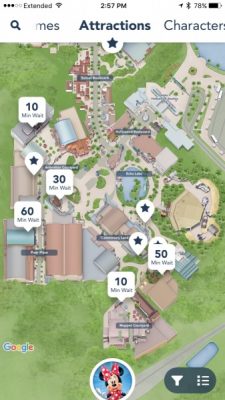This screenshot from a smartphone displays a navigation interface for a theme park, likely Disney World given the presence of a Minnie Mouse icon. The background is predominantly white with a central top display showing the time as 2:57 p.m. and a battery level at 78%, positioned to the right. Below this, a search bar with a magnifying glass icon is labeled "attractions", and adjacent to it is the word "CHARACTER" in uppercase letters. 

Further down, a map is visible against the same white background, showcasing various areas within the park, characterized by green spaces. The map includes icons for different rides, each annotated with waiting times, such as 10 minutes, 30 minutes, and 60 minutes. Certain attractions are highlighted with stars. The bottom of the screen features an image of Minnie Mouse, reinforcing the Disney World theme park setting.